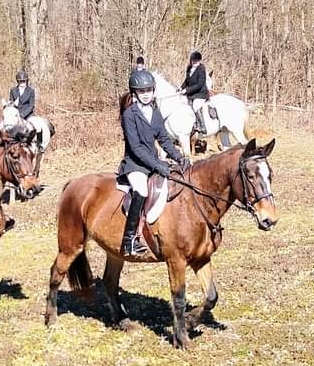This photograph captures an outdoor scene featuring four riders on horseback, positioned in a grassy, wooded field with a mix of browns and sparse greenery, suggesting late fall or early winter. The primary focus is a young girl riding a small brown horse. She is dressed in traditional English riding attire, complete with a black riding jacket, black hat, white riding pants, and black boots. Her hair is neatly pulled back into a pigtail, and she’s seated on an English saddle. The brown horse she rides has distinctive black markings on its legs and is standing with one leg slightly bent. Behind her, another brown horse's head is partially visible, although its rider is not. Further back, a white horse is ridden by an unidentified individual also dressed in English riding gear. The background shows two more riders on white horses, though they are less prominently visible. The overall setting is calm, with the horses standing still against the muted backdrop of the field and sparse trees.